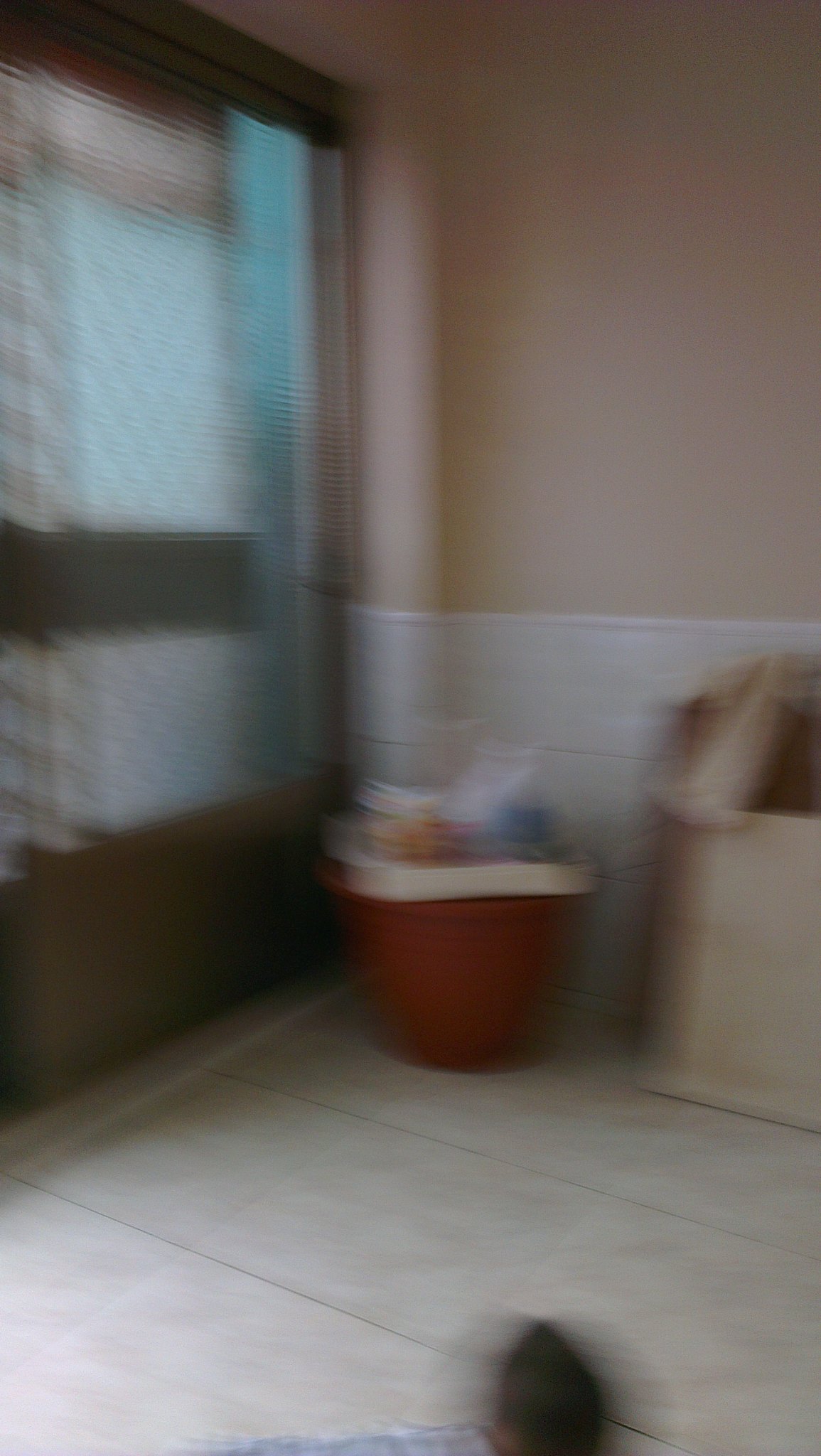This image appears to be a very blurry photograph of an interior space that is not residential. The floor is covered with large, square, whitish tiles that extend halfway up the walls. Above the tiles, the walls are a light pinkish or flesh color. In the center, up against one of the walls, there is a round column covered in the same tiles as the floor and lower walls. 

A significant feature in the back corner of the room is a large, reddish-orange pottery planter with indistinct objects, possibly packages, on top of it. To the left, a wall with a tall window covered by light blue curtains can be seen, although it’s unclear whether they are pulled aside or fixed. On the right side, there's a larger, possibly cardboard box. Additionally, the image captures what seems to be a person's leg and foot at the bottom center, hinting at some human presence, although due to the blurriness, it's indistinct.